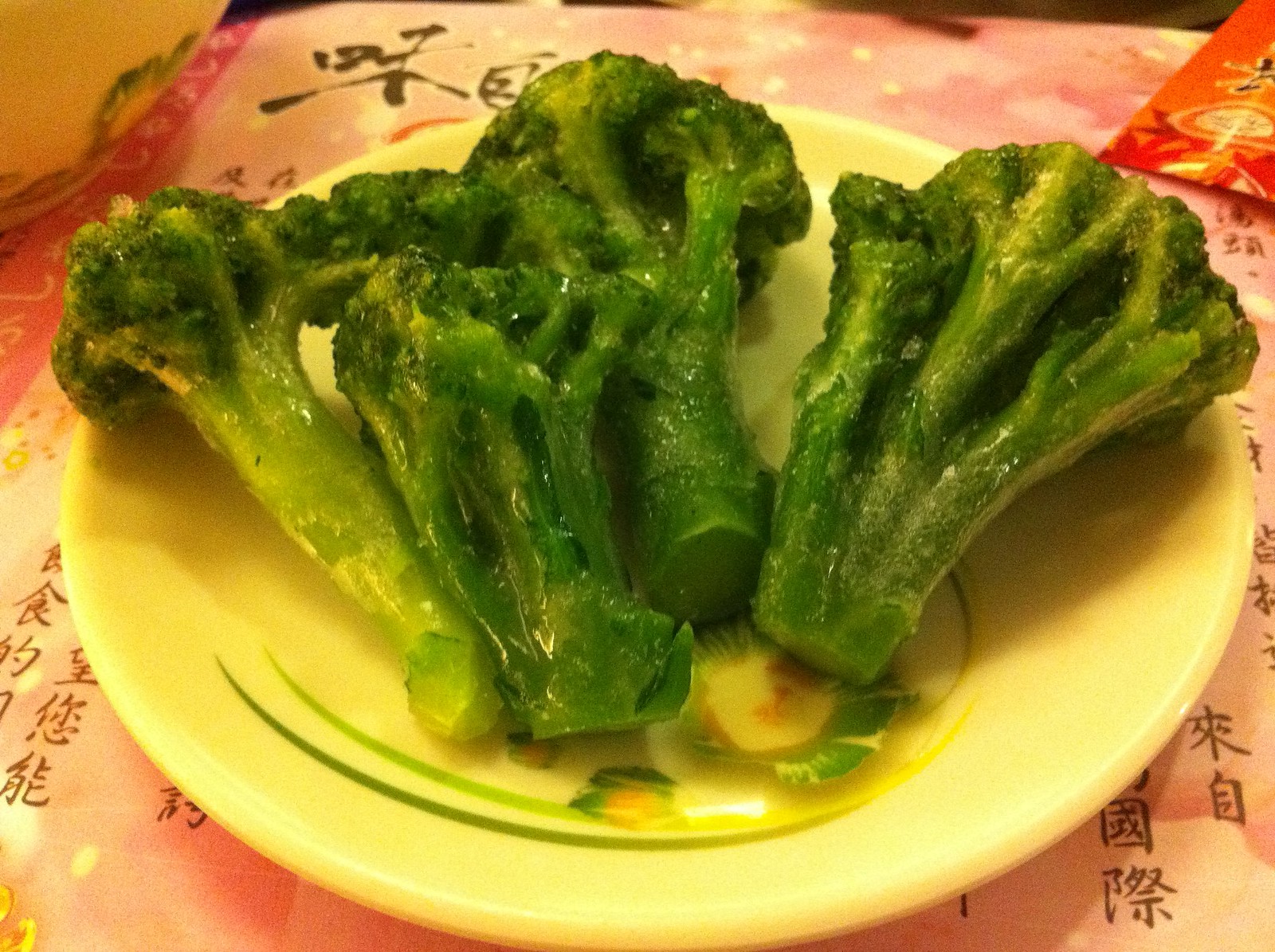A vivid and somewhat unappetizing plate of broccoli is displayed on a light yellow plate adorned with a yellow flower and green lines at the bottom. The broccoli appears overcooked and limp, but still retains a glowing, vivid green color, possibly glazed with a shiny, clear butter sauce. There are five small pieces of broccoli arranged in an arc on the plate. The plate itself sits on a red tablecloth featuring black Chinese script, adding a contrasting backdrop to the scene. In the top right corner of the image, there is a paper tube containing chopsticks, suggesting a restaurant setting. The vibrancy of the green broccoli against the colorful, ornate dish and the red tablecloth create a striking visual, albeit the broccoli itself looks less appealing.